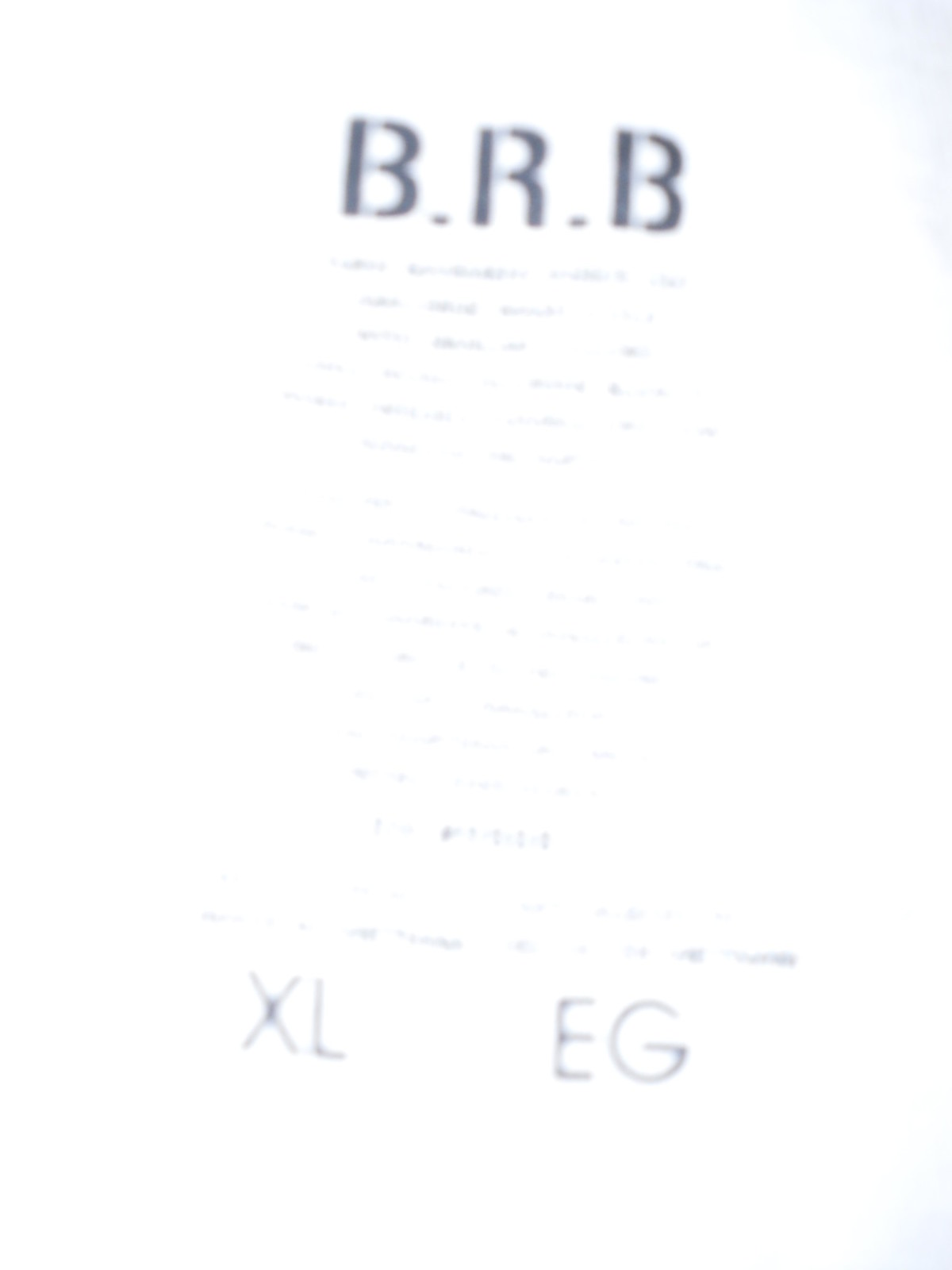This image showcases a faint and slightly blurred piece of paper. The overall tone of the image is quite dull and light, making it challenging to discern specific details. At the top center of the paper, there are gray letters that read "B. R. B." with a period after each letter. The middle portion of the paper contains some writing, but it is largely unreadable due to the blur and dullness of the image. As you move further down the paper, the text becomes marginally clearer although it remains difficult to read. The bottom of the paper features a distinct line of text that is easier to make out, though still not entirely clear. Flanking this clearer text, there are two sets of letters: "XL" on the left and "EG" on the right.